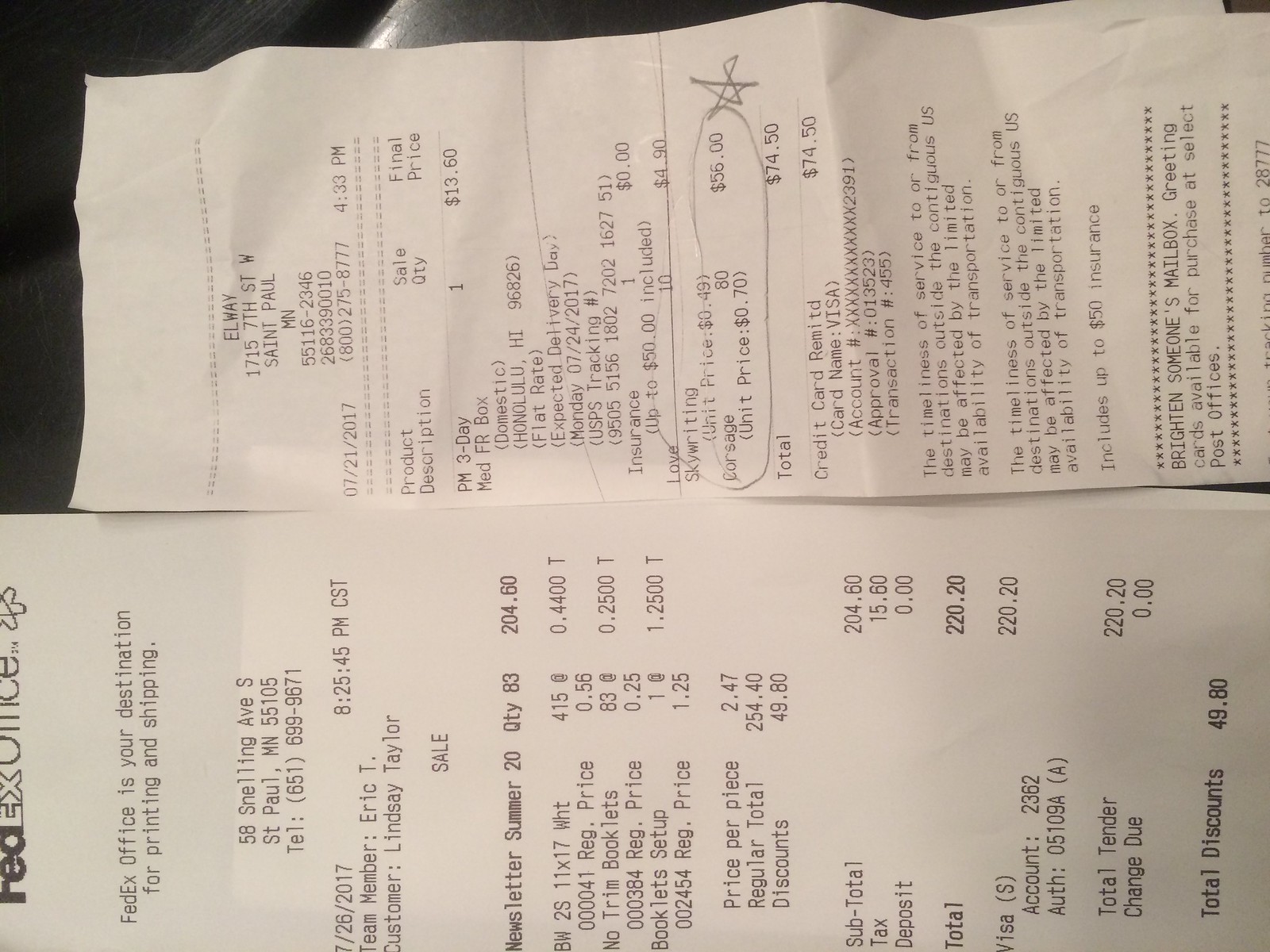This close-up photograph showcases two horizontally-aligned receipts, requiring a head tilt for proper viewing. Both receipts are from different vendors in St. Paul, Minnesota and are dated around the same period in late July 2017.

The first receipt, positioned at the bottom, is from FedEx Office located at 58 Selling Avenue S, St. Paul, MN 55105, with a contact number 651-699-9671. Detailed information includes the purchase time of 8:25 PM CST on 7-26-2017. Items listed include newsletters (summer 20) in a quantity of 83, BW2S 11x17 white paper with no trim booklets, and booklet setup. The initial total was $254.40, but after discounts of $49.80, the final amount came to $220.00, paid via Visa card.

The second receipt, situated on top, is from Elway also in St. Paul, dated 7-21-2017. A notable detail is a circled expenditure labeled “skywriting” amounting to $56.00, marked with an asterisk. Additional purchases include a PM 3-day Med FR box priced at $13.60 and another insured package. The total expenditure on this receipt is $74.50, again paid using a Visa card.